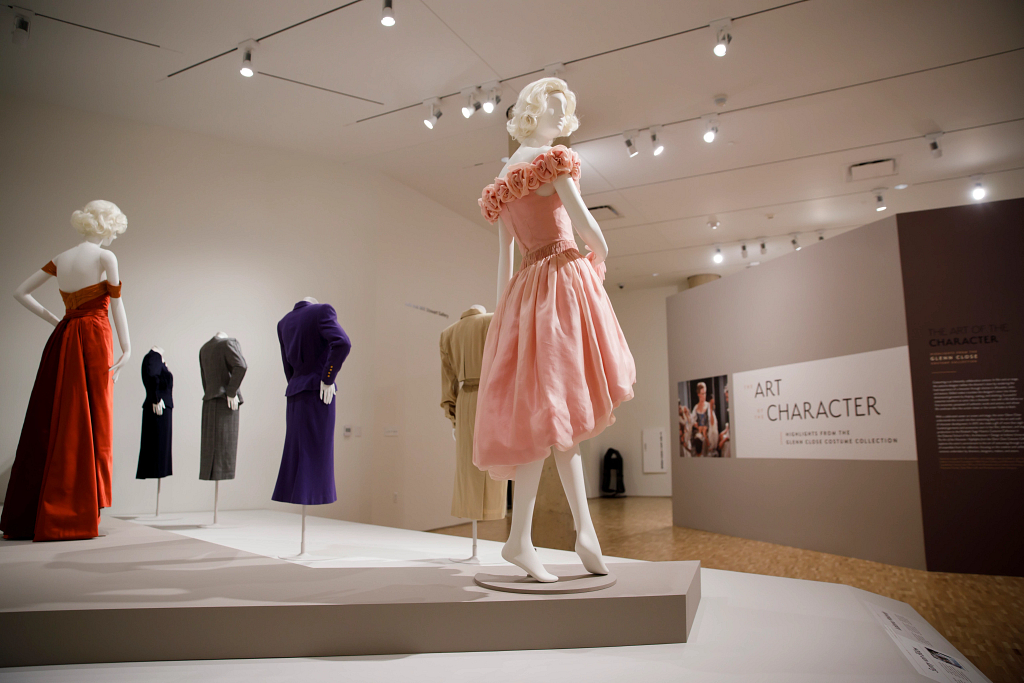Inside a spacious, white-walled museum or fashion exhibition, an array of mannequins are prominently displayed on a raised beige platform that dominates the left side of the room. In the foreground, one mannequin with white skin and blonde hair dons a luxurious, off-the-shoulder, floor-length red satin dress, giving it an air of elegance. Nearby, another mannequin, also white-skinned and blonde, showcases a pink, mid-length dress adorned with rosette detailing around the bodice, which rises slightly higher in the front than the back.

Centered behind these mannequins are four headless and legless dress forms, each wearing a similarly styled outfit in different colors: a deep purple suit and dress, an army green suit and dress, a dark gray suit and dress, and a black suit and dress. These dresses appear quite plain and formal, suggesting office attire.

To the right side of the exhibit, a panel reads "Art of the Character," accompanied by a slightly blurred image of an actress that seems to depict a movie scene. This photograph hangs on the left side of the panel, reinforcing the theme of character-focused art and fashion within this thoughtfully curated space. The room’s ceiling is wide and triangular, adding to the modern, clean aesthetic of the exhibition.